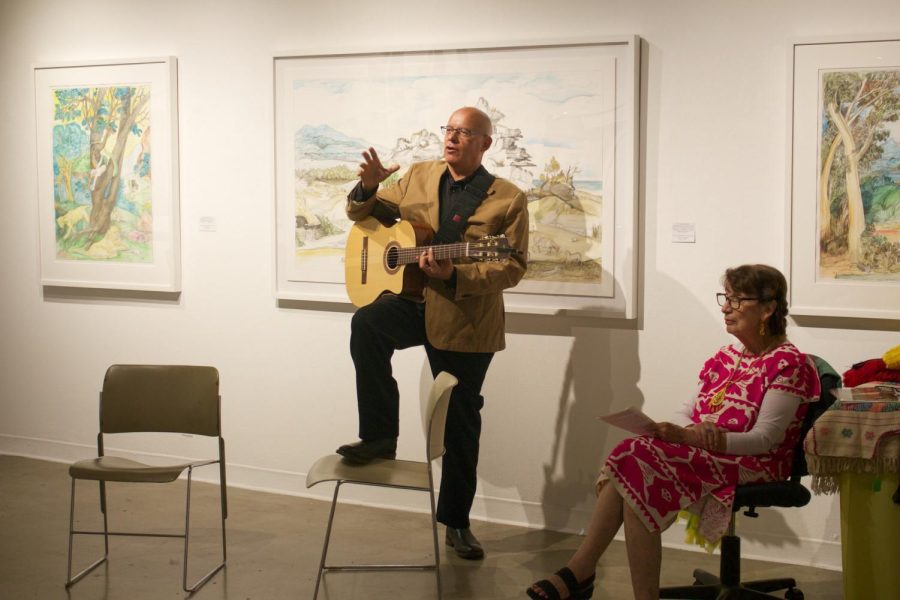In this indoor photograph, a bald man stands prominently in the center with his right leg resting on a wooden school chair. He is wearing black boots, black pants, and a brown jacket over a black shirt. The man is in the middle of speaking, raising a hand out in front of him, while the other hand is poised to strum a guitar that is strapped around his shoulder. Behind him, the white wall showcases three pieces of artwork with what appears to be a label between them. To the left of the man, a woman is seated in an office chair. She is wearing glasses and a red and white dress, holding a piece of paper in her left hand and wearing sandals. The scene captures the man engaging with his audience, possibly in an artistic or educational setting.